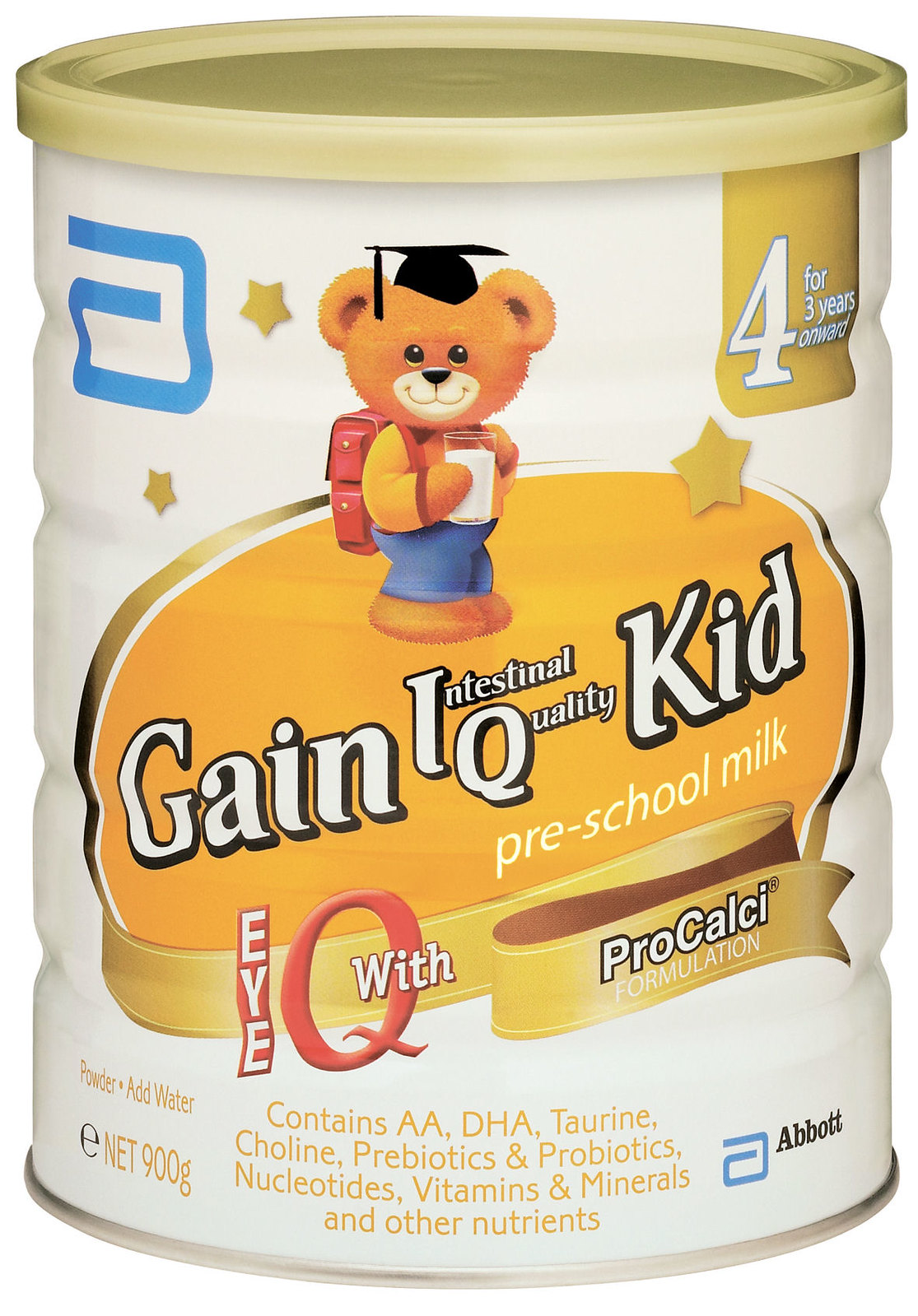The image is an advertisement for a can of preschool milk, prominently marked as "Gain Intestinal Quality Kid Preschool Milk." The packaging features a colorful and detailed design with a yellow lid and a white cylindrical body. At its center, enclosed in an orange oval, are the words "Gain Intestinal Quality Kid." Underneath, the product is labeled "Preschool Milk." A backwards "G" with two stars adorns the upper left corner. 

A cute, cartoony bear character is depicted, wearing a graduation cap, red backpack, yellow shirt, and blue pants, and holding a glass of milk. To the right of the bear, there's a star and a banner stating "4 for 3 years onward." 

A gold ribbon on the packaging displays the "IQ, EYE-Q, and Pro Cal C formulation" text. The bottom part of the can lists the inclusion of beneficial nutrients such as AA, DHA, Taurine, Choline, Prebiotics, Probiotics, Nucleotides, Vitamins, and Minerals. The can weighs over 900 grams and is manufactured by Abbott.